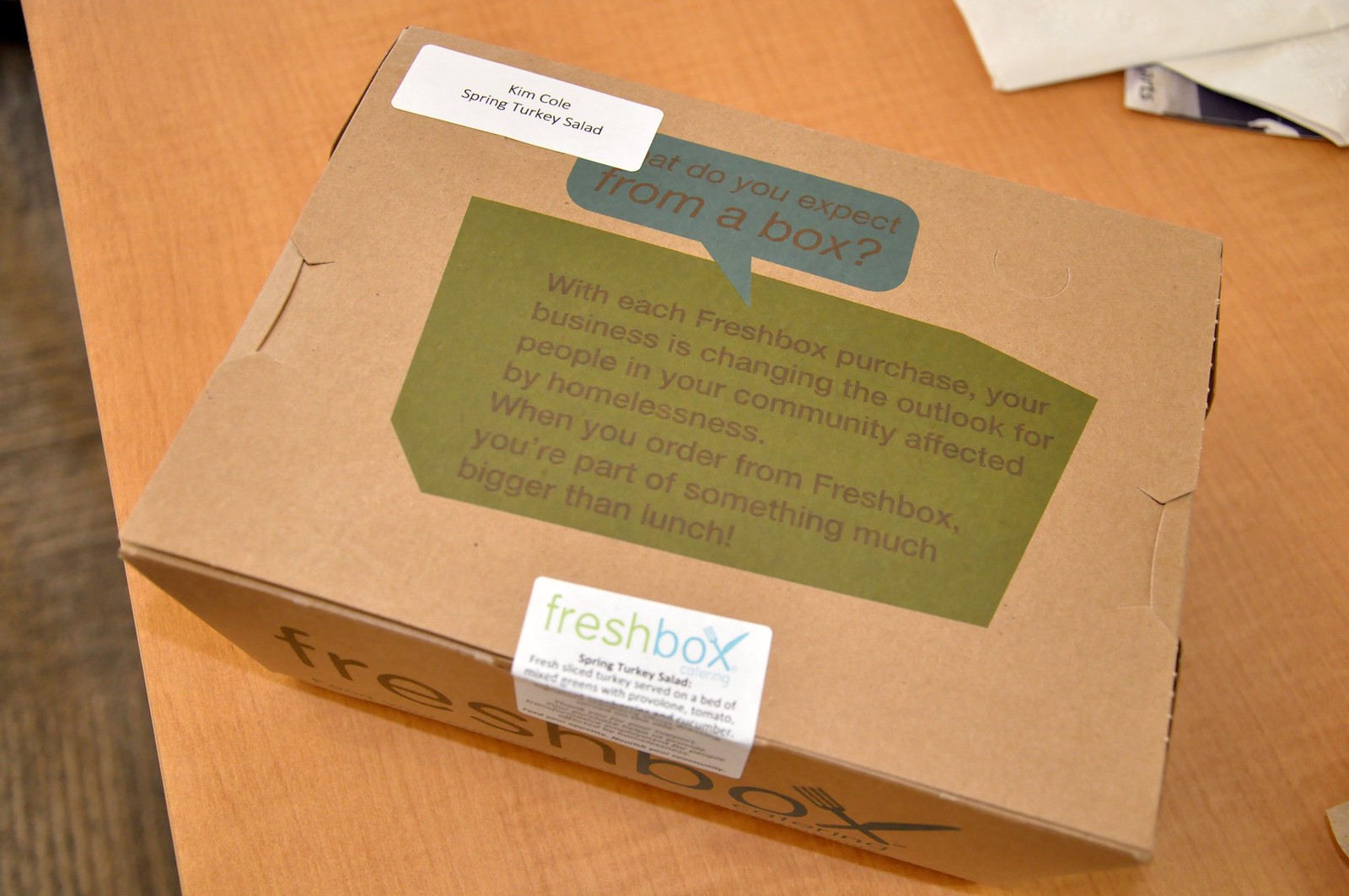The indoor photograph captures a cardboard package placed on a wooden table with a bit of brown carpet visible on the left side. The box prominently features a white sticky label on the upper left-hand side that reads, "Kim Cole Spring Turkey Salad." In the middle of the box, set against a green background, the text in black font says, "With each fresh box purchased, your business is changing the outlook for people in your community affected by homelessness. When you order from FreshBox, you're part of something much bigger than lunch." The side of the box displays the brand name "FreshBox," with the 'X' represented by a crossed fork and knife. Additionally, there are a few white papers and one paper with blue accents near the upper right corner of the table.